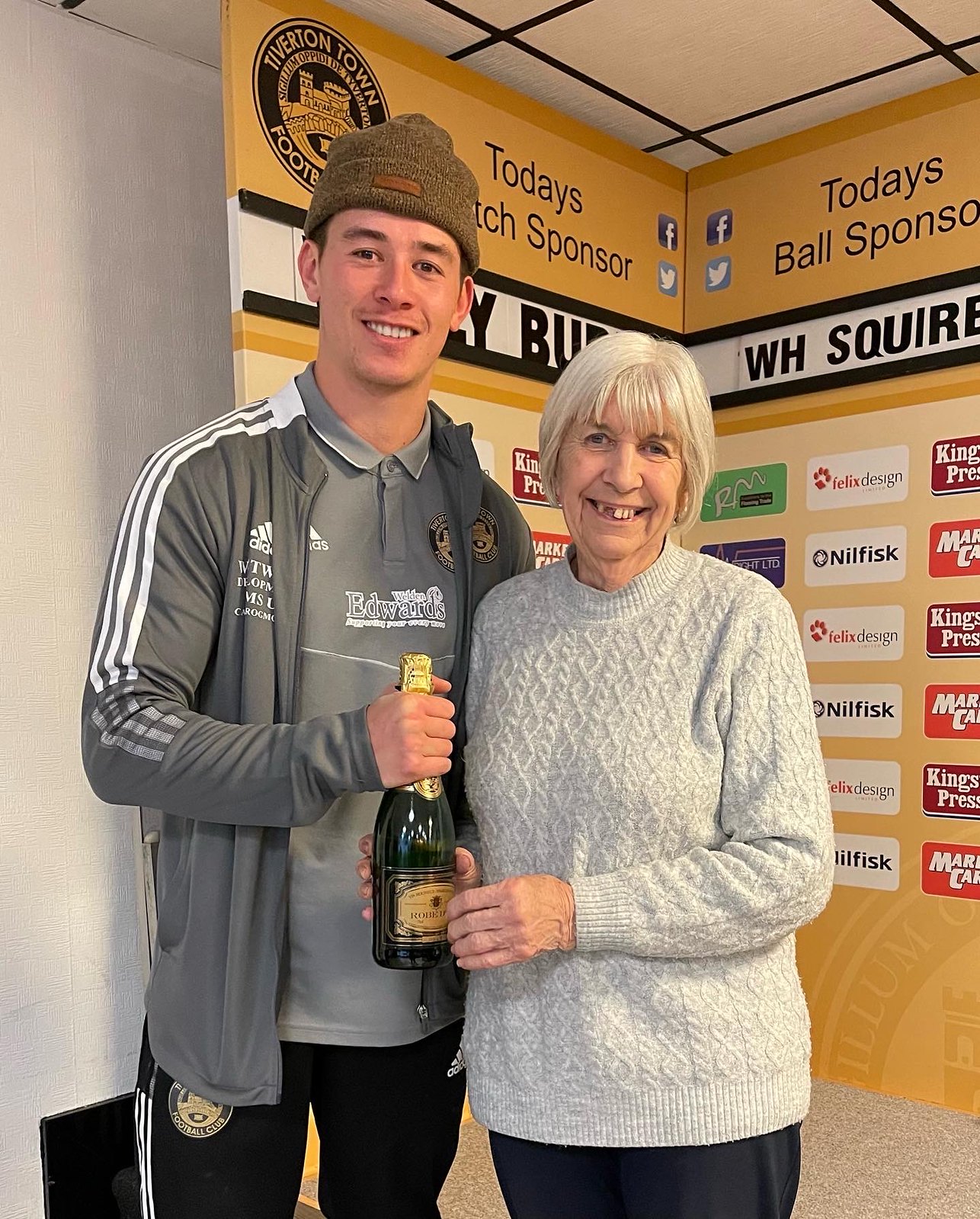In this indoor photograph, a young man and an elderly woman are posing together in front of a cardboard stand that reads "Today's Ball Sponsors," with various sponsor names and logos, including Neal Fiske. The young man, positioned to the left, is much taller and is wearing a gray Adidas jacket and pants, along with a brown beanie. In his right hand, he holds a bottle of champagne or wine, which the elderly woman also holds at the base. The woman, standing to his right, has shoulder-length white hair, a couple of missing front teeth, a gray sweater, and dark pants. Both appear to be smiling for the camera. The background displays logos of social media platforms like Facebook and Twitter, and other sponsor logos, although some are partially cut off by the edge of the photograph. The walls behind them are yellow and form a corner. The setting and signage suggest the photo may have been taken at a soccer event organized by the Tiverton Town Football Club.